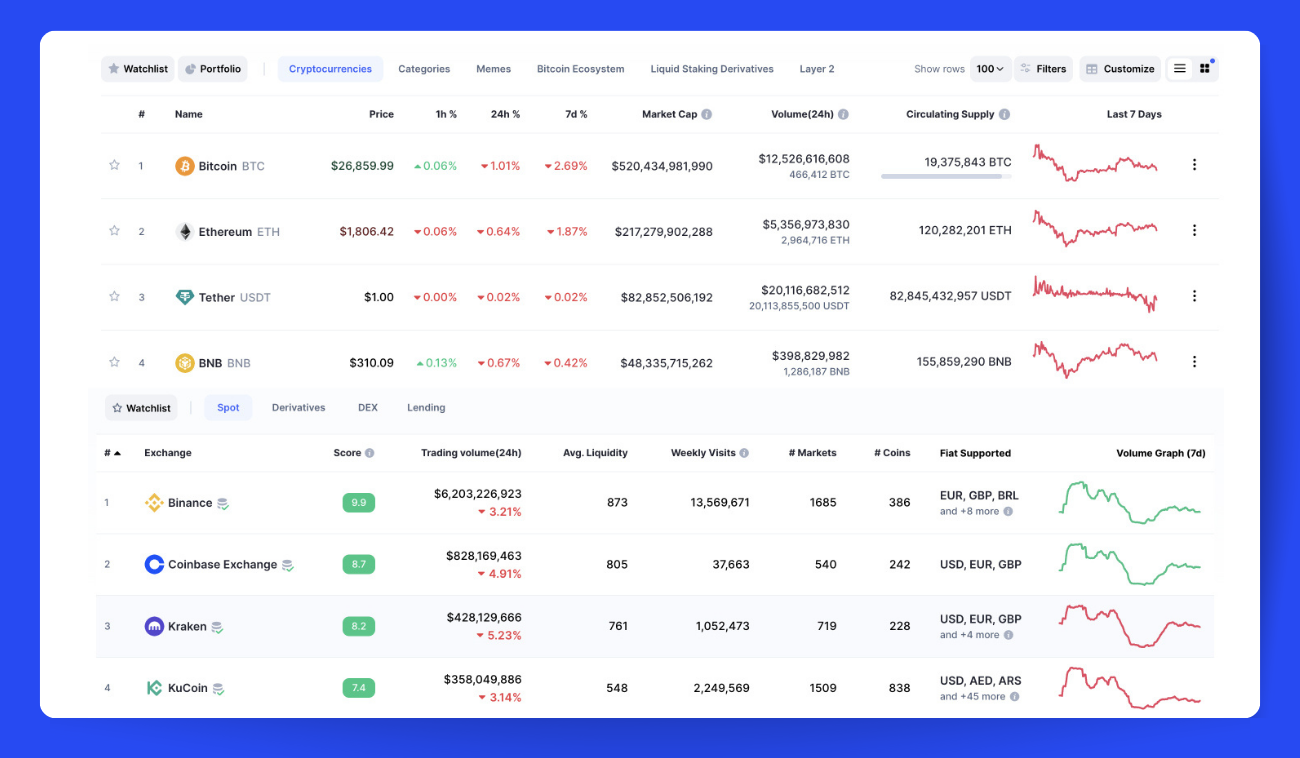The image depicts a comprehensive financial dashboard on a white background framed by a thick blue border. At the top, there are options labeled "Watch List", "Portfolio", "Cryptocurrencies", "Categories", and "Memes", although the last tab is difficult to discern due to small text size. The dashboard features various financial statistics, presented in sections with organized data.

Key elements include:
1. A prominent "180" number within a blue box, followed by another similar box.
2. Three horizontal lines and a set of four small black squares each topped with a blue dot.
3. Listings for different assets such as Bitcoin, Ethereum, Tether (USDT), and Binance Coin (BNB), each accompanied by respective prices and relevant statistical data.
4. Small graphs illustrating price trends over the last seven days, with notable red numbers indicating downturns.
5. A blue underline highlighting the "Circulating Supply" of one asset.
6. Categories for different exchanges, each paired with green boxes that display numeric values.
7. At the end of several rows, additional graphs depict upward and downward trends.

The dashboard integrates a variety of visuals and numeric data for easy monitoring of financial and cryptocurrency markets.